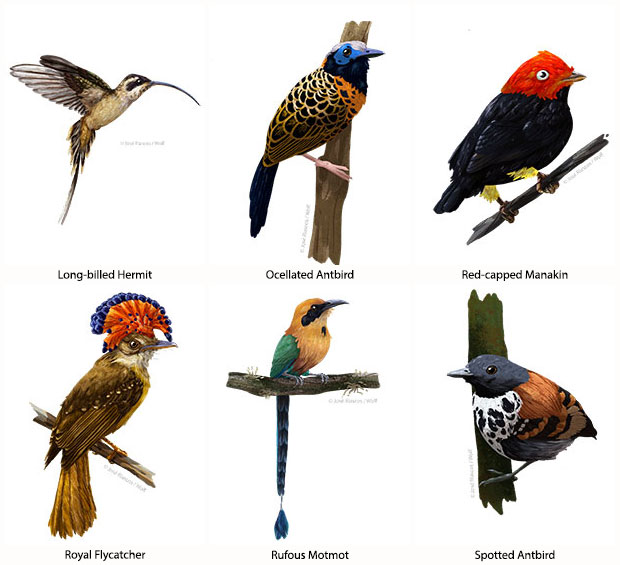The image features detailed drawings or paintings of six diverse bird species arranged in two rows of three. The top row includes: the long-billed hermit, characterized by its needle-like curved beak and small body, depicted in flight; the oscillated ant bird, notable for its blue head and neck, dark neck, orange breast, and black and yellow body; and the red-capped mannequin, easily identified by its striking red head and black body. The bottom row showcases: the royal flycatcher, with its distinctive brown body and an elaborate fan-like crown of orange with blue tips; the rufous motmoth, featuring a green body, a golden breast and head, and green wings; and the spotted ant bird, which has a blue head and neck, a white crest with black spots, a yellow and black spotted belly, and brown wings. All birds, except for the long-billed hermit in flight, are perched on twigs or small branches.